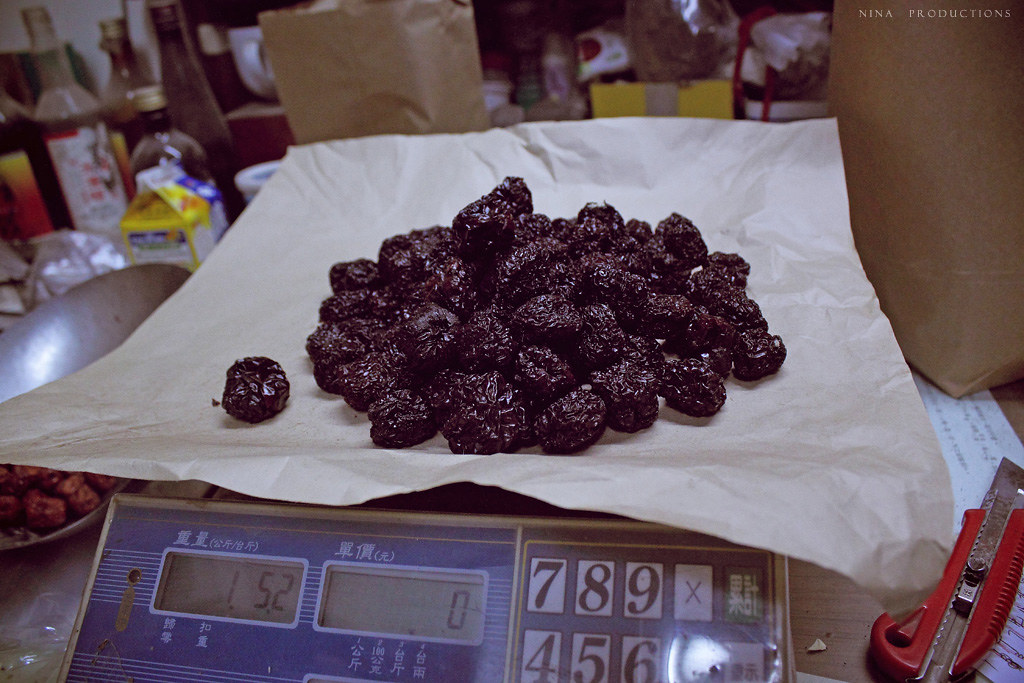The photograph captures a detailed scene centered around a digital scale, likely situated in an open-air market or a modest shop. On the scale, which might be of Chinese or Asian origin, there is a pile of wrinkly dried fruits, potentially jujubes or dates, placed on a piece of paper. The scale's digital display reads "1.52" on the left and "0" on the right. The scale also features a partly visible keypad with numbers 7, 8, 9, 4, 5, 6, and an "X," accompanied by some Asian characters. To the right of the scale, a red-handled box cutter knife rests on the table. Surrounding the central setup, there are paper bags, open bottles, and a jumbled assortment of items, suggesting a busy, cluttered environment. The top right corner of the image mentions "Nina Productions."